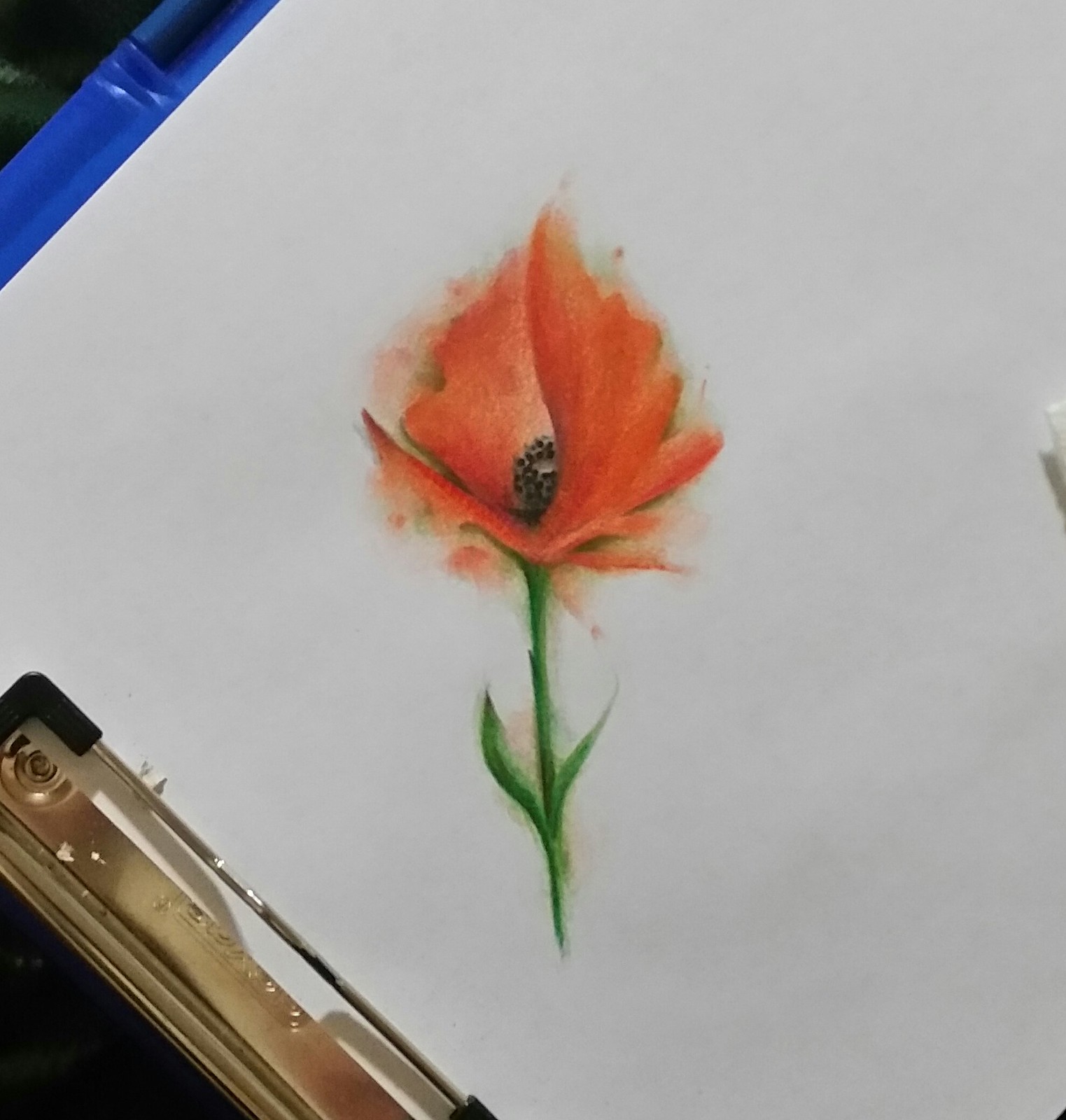The image features a piece of white paper clipped securely to the left-hand side of a clipboard, visible at the bottom left corner with a silver-toned clip and black plastic brackets. In the center of the paper, there's a colored pencil drawing of a flower. The flower has large, irregularly shaped scalloped petals, which are primarily light pink with hints of red and orange, giving them a delicate and almost dripping appearance. At the heart of the petals lies a small gray and brown seed pod or cone-like structure. The dark green stem, adorned with spiky leaves at its base, extends from the bottom middle to the top middle of the paper. Additionally, a blue pen, likely the barrel, rests atop the paper in the upper left corner, adding a touch of extra detail to the composition.